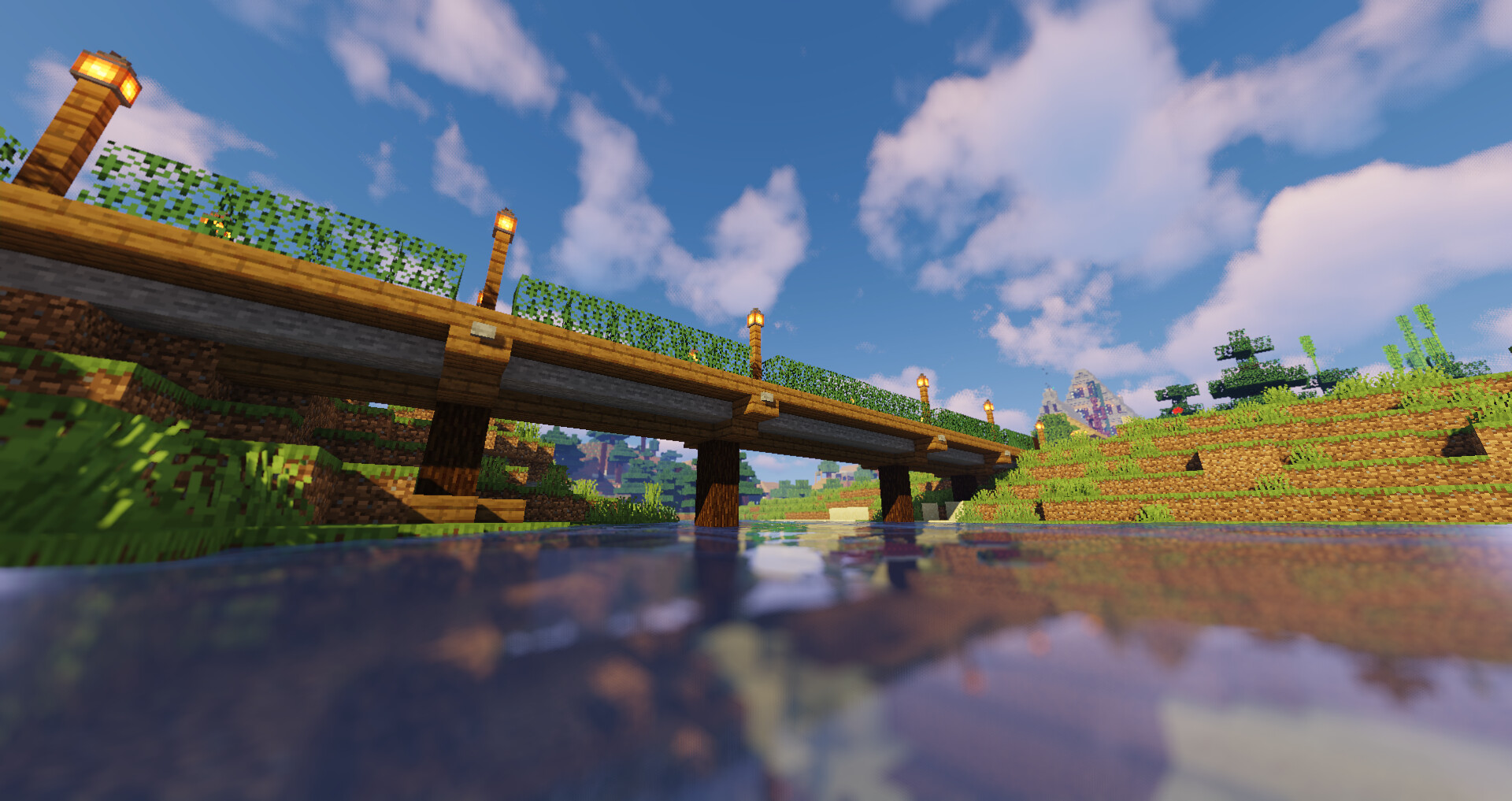The image is a detailed, still capture from a video game, likely Minecraft or a similar block-based game. It presents a serene vista overlooking a body of water. A meticulously crafted bridge extends across the water, composed of brick cubes with sections ascending towards illuminated posts made of fire cubes at regular intervals. The terrain, characterized by its cubic composition, includes brown rocky dirt and lush green grass cubes. In the background, a hill made from the same blocky terrain rises from the edge of the water. Above, the sky boasts a brilliant blue hue, dotted with fluffy white clouds, adding a sense of calm and tranquility to the pixelated landscape.